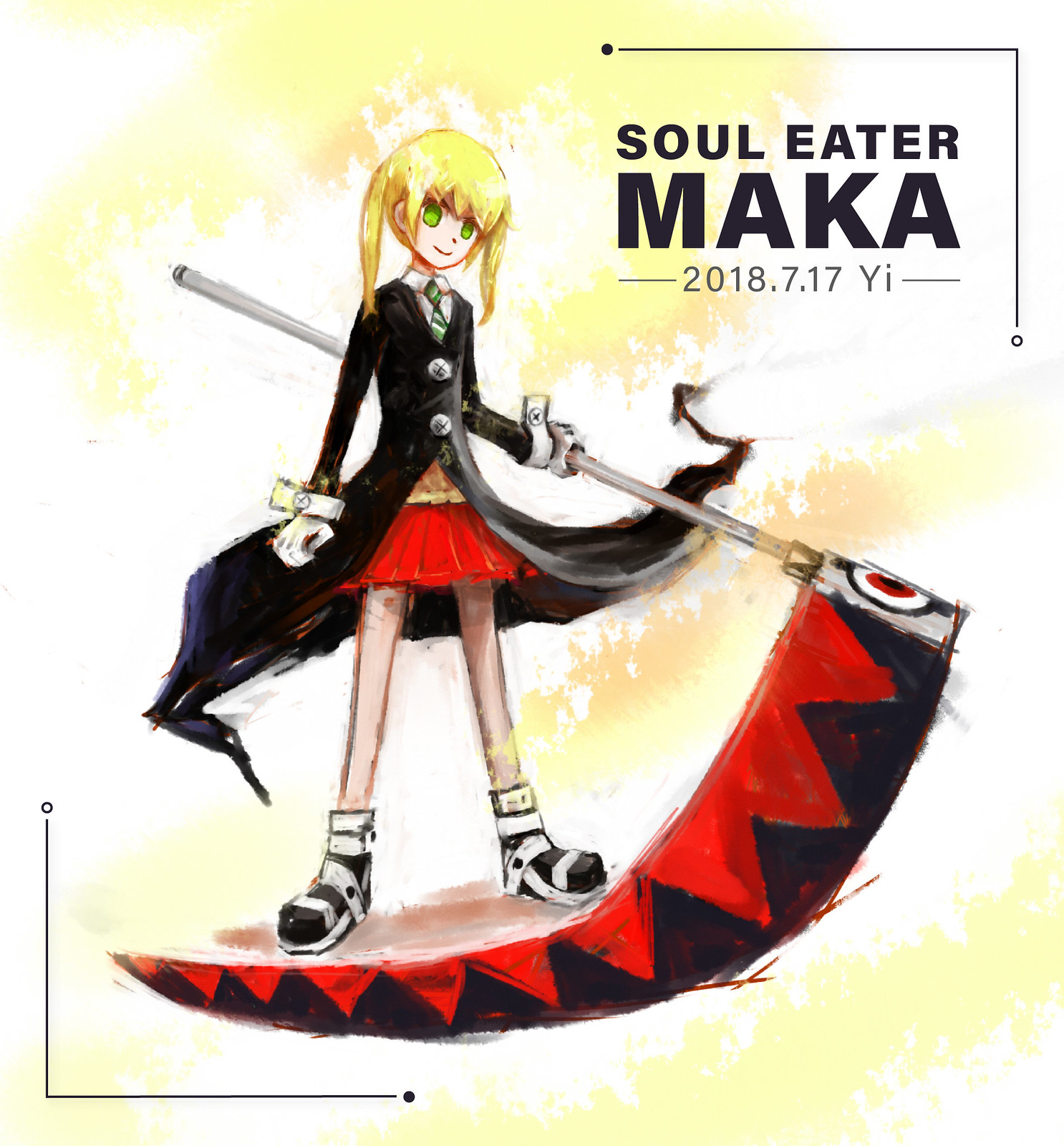This is a detailed, full-color print piece featuring a hand-drawn anime character standing centrally against a primarily white background with subtle yellowish accents. At the top right corner, the image is captioned with black text reading "SOUL EATER" and "MAKA" in bold, all-caps. Below this, the date "2018-7-17-YE" is displayed. The character depicted is a young girl with short blonde hair and striking green eyes. She is dressed in a black jacket with gray buttons and a green tie over a white shirt, paired with a very short red skirt. She accessorizes with a gold belt and wears black and white boots. The girl brandishes a large, red and black scythe reminiscent of the Grim Reaper's weapon, indicating her formidable nature. The scythe features a black shaft adorned with red triangular patterns. The composition of her attire, along with the flowing lines of her jacket or skirt, adds a sense of dynamic movement to her pose.